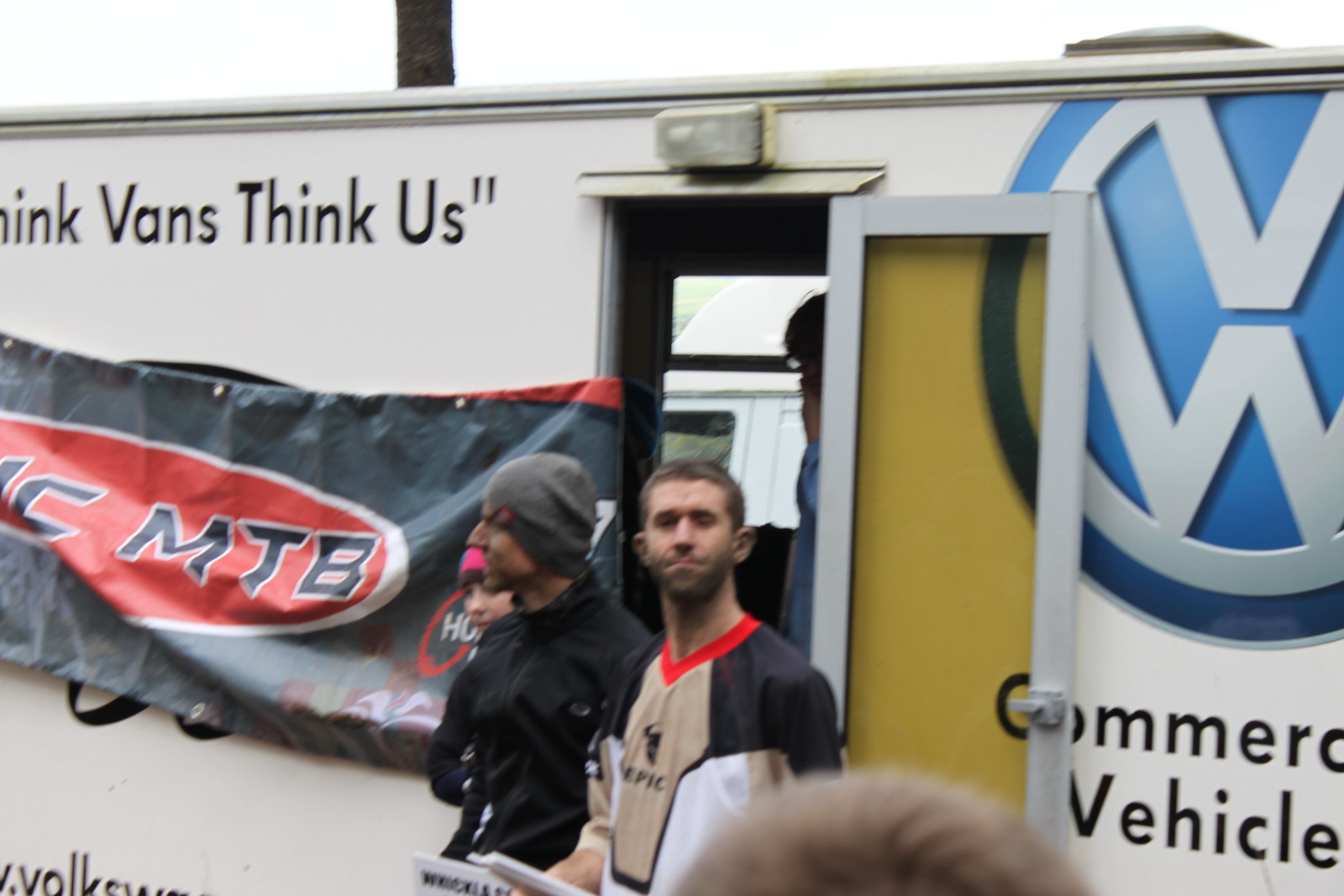The image is a somewhat blurry outdoor photograph capturing a white trailer with a prominent blue and white Volkswagen logo and the words "commercial vehicle" written below it. The trailer has an open door with yellow-tinted glass, and inside, a person is partially visible. Outside the trailer, three people are standing in the foreground. The first person, a white male with brown hair and stubble, is wearing a practice soccer jersey. Next to him is a man in a black jacket and gray beanie. The third figure is less distinguishable but could be either a child or a woman. Additionally, the trailer displays a banner with a red background and "MTV" written in white and black. The scene also includes two more individuals faintly visible in the background.